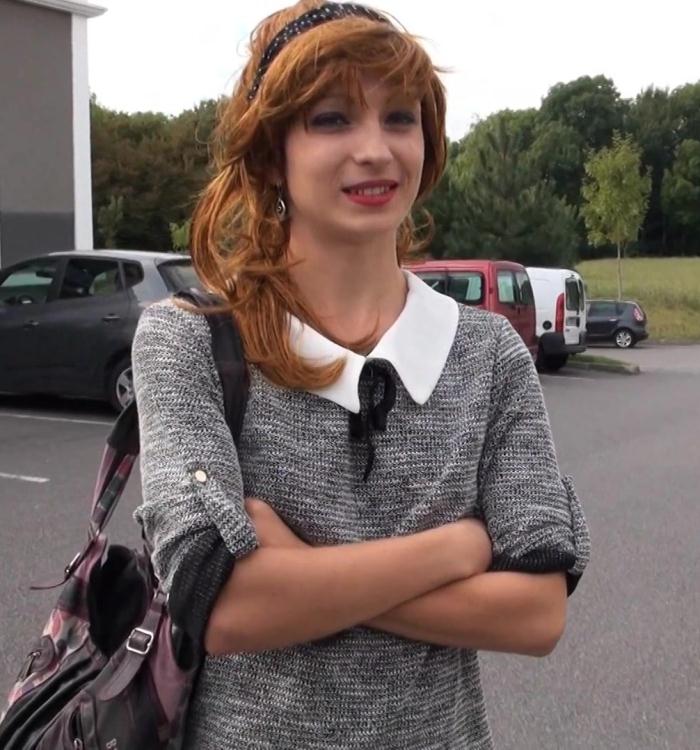In this close-up color photograph taken outside in a bustling parking lot, a young woman, approximately 20 years old, stands confidently. Her long, slightly wind-tousled hair is a striking blend of red and brown, held back by a distinct black headband adorned with white dots. She wears red lipstick that complements her outfit—a gray and white tweed dress with a classic white collar and a black bow tied in front. The dress resembles a sweater, adding to its cozy appearance. Around her right shoulder is a striking purse with colors of purple and black, and her arms are crossed neatly in front of her chest. In the background, a variety of cars—black, red, white, and more—are lined up in the parking lot. Behind these vehicles, a stretch of lush green grass and a forest of trees under a white sky complete the serene setting.